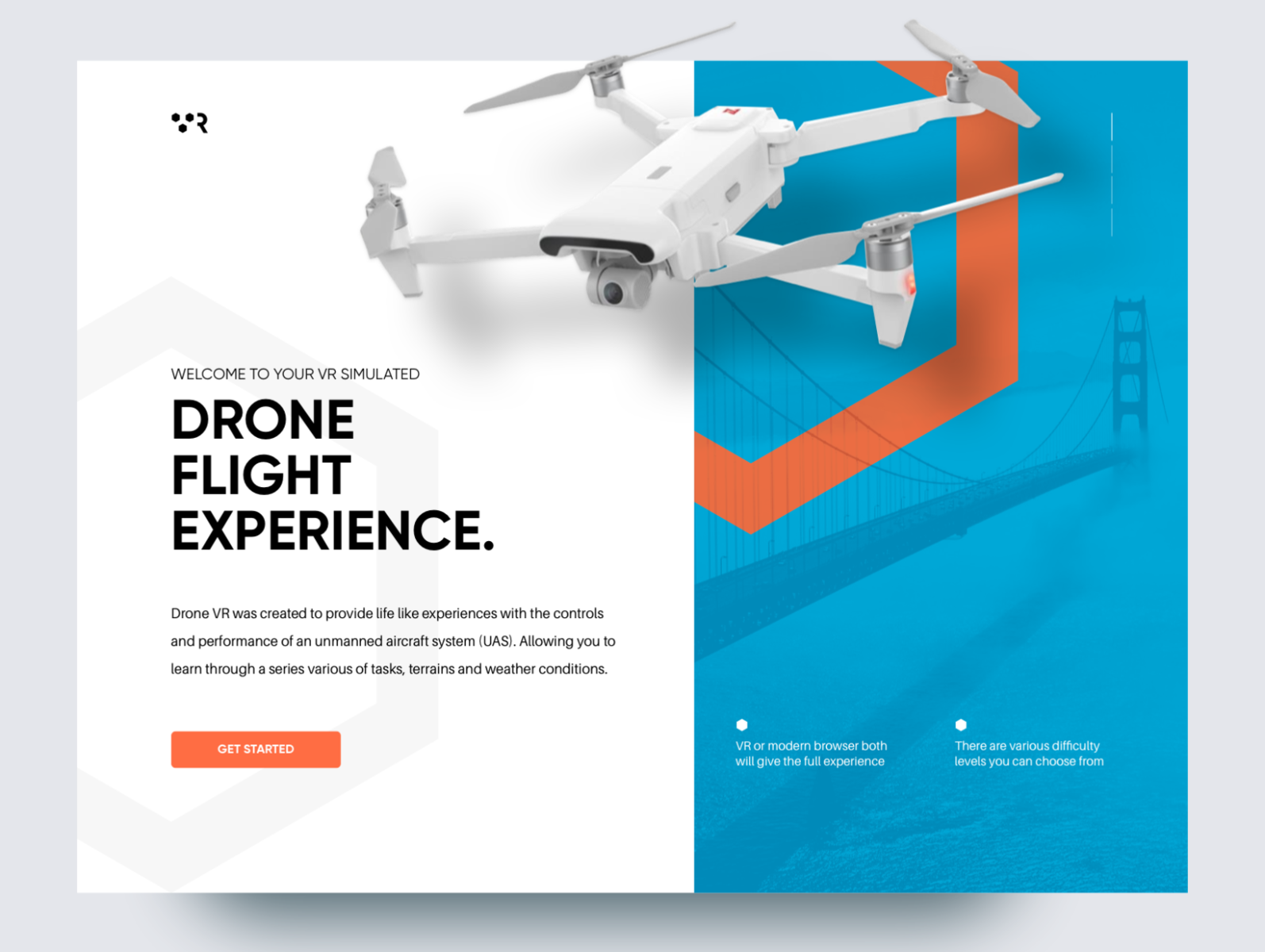The image depicts a cropped section of a website's landing page with a light gray background. Central to the image is a square divided into two sections: approximately 60% on the left features a white background, while the remaining 40% on the right is ocean blue. The blue section subtly showcases the Golden Gate Bridge in the background.

Overlaying the blue area is an orange octagonal symbol, reminiscent of a stop sign, containing white text at its bottom area. Positioned at the juncture of the blue and white halves, a white drone is prominently displayed.

To the left of the image, the text reads: "Welcome to your VR simulated drone flight experience. Drone VR was created to provide lifelike experiences with the controls and performance of an unmanned aircraft system (UAS), allowing you to learn through a series of various tasks, terrains, and weather conditions."

At the bottom-left corner, there is an orange button labeled "Get Started."